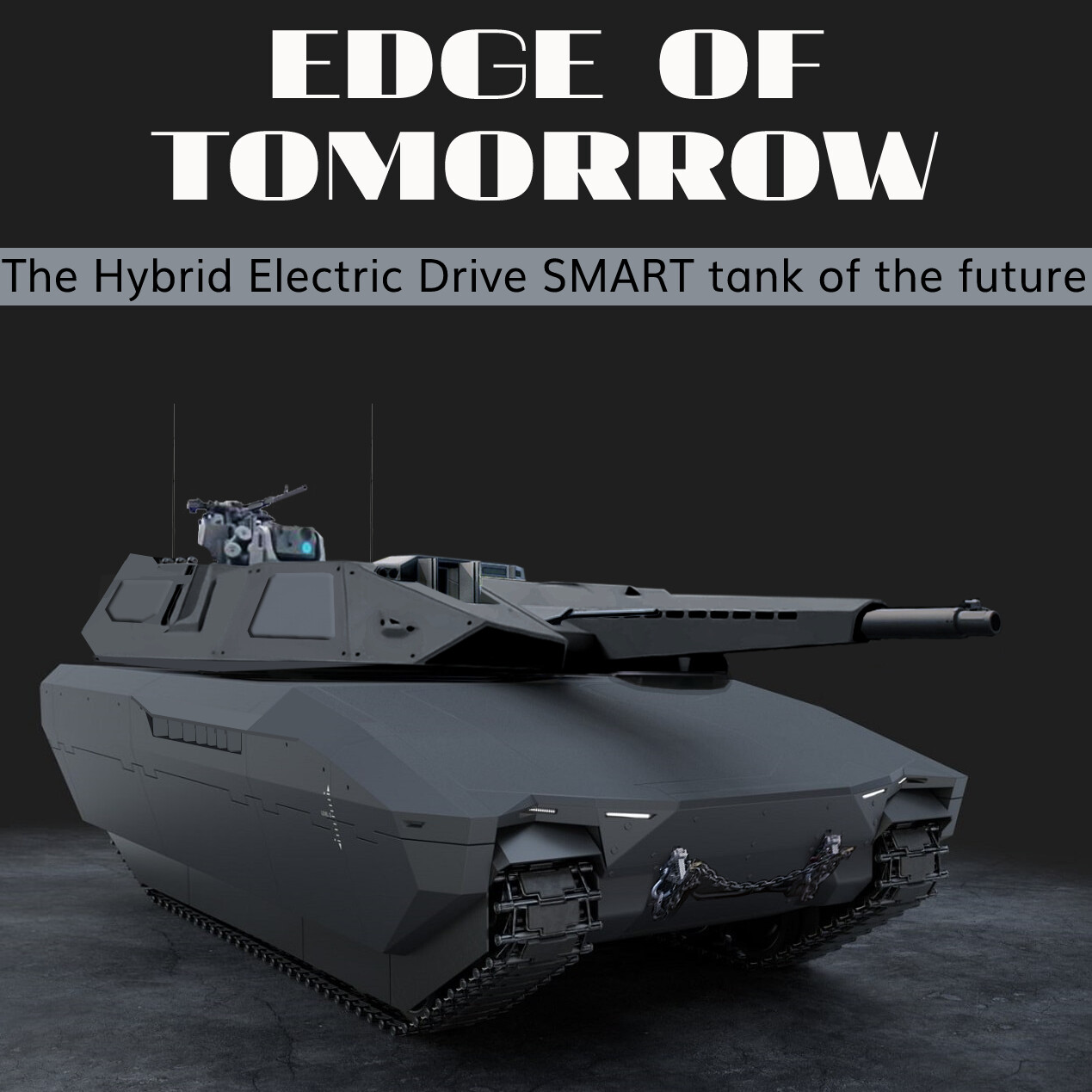This image appears to be an advertisement, featuring the headline "EDGE OF TOMORROW," written in bold white typography against a solid black background. Below this, a light gray band contains the tagline "The Hybrid Electric Drive Smart Tank of the Future," with the word "SMART" emphasized in all capital letters. The primary focus of the image is a highly detailed, sleek, and futuristic tank. Unlike traditional tanks with rounded edges and visible mechanical components, this one boasts smooth, polygonal lines that resemble the stealthy design of a sports car or a stealth bomber. Its color scheme is a cohesive, dark black and gray, complementing the overall modern and advanced aesthetic. The tank is equipped with a prominent large gun at the front and what appears to be a smaller gun or possibly an electronic device at the rear. The tank's treads are visible, reinforcing its grounded functionality despite the futuristic design elements. The entire composition rests on a simple black and white surface, highlighting the tank's innovative design in the context of a stark, minimalistic environment.